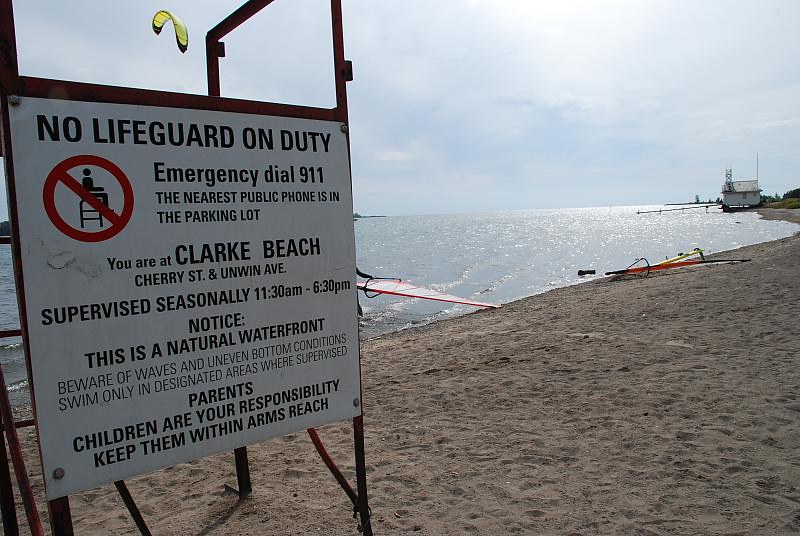This image captures a serene beach scene at Clark Beach, located at Cherry Street and Unwin Avenue. The sandy shoreline extends to the right, meeting the calm blue water on the left. Above, a clear sky with scattered clouds stretches across the horizon. In the foreground, a prominent white sign with black text, mounted on a metallic post, alerts visitors that there is "No lifeguard on duty." The sign provides crucial safety information, instructing in case of emergency to dial 911 and directs to the nearest public phone located in the parking lot. It highlights that the beach is only supervised seasonally from 11:30 a.m. to 6:30 p.m., warns about the natural waterfront conditions, and emphasizes parental responsibility for children's safety. Behind the sign, a yellow parachute from a hang glider is visible, partially obscuring the hang glider. The scene is bathed in warm sunlight, creating a peaceful yet cautious coastal atmosphere.